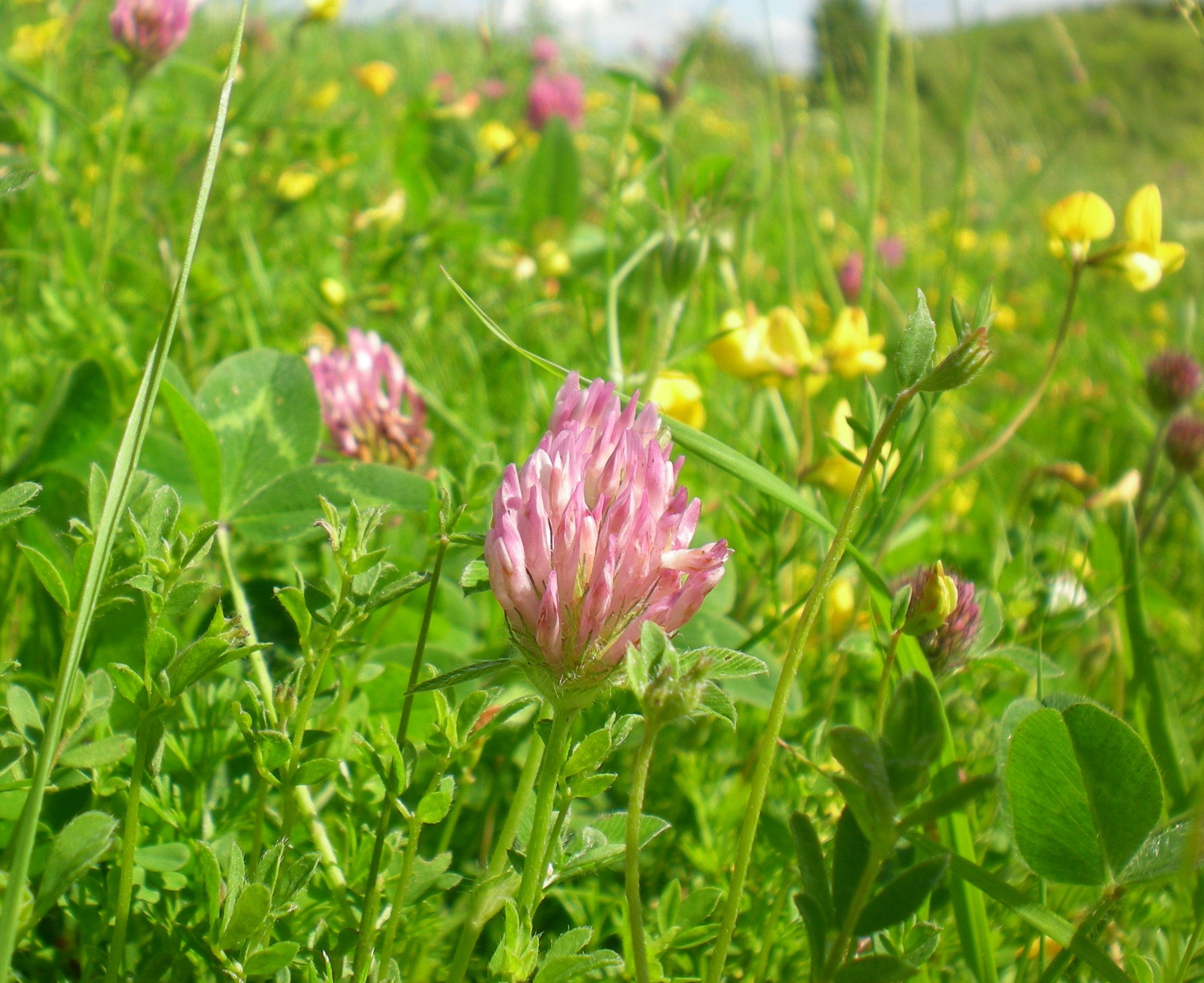This vibrant and detailed photograph captures the lushness of a sunlit field blanketed with a variety of flowers and rich greenery. Dominating the scene are light lavender flowers reminiscent of purple clovers, standing resiliently on robust stems adorned with larger leaves. Interspersed among these are yellow flowers, possibly resembling buttercups with their small, lily-like petals atop slender green stems. The field itself is a tapestry of medium to dark greens, with blades of grass protruding through the floral display, enhancing the textural variety. In the blurred background, hints of bright blue sky peek through, adding depth to this picturesque natural landscape. The close-up perspective highlights the vivid brightness of the greenery, almost yellowish in its radiance, contrasting beautifully with the pink buds of partially open flowers that resemble red clovers. Smaller buds and the tall grass in the foreground further contribute to the intricate mosaic of colors and forms, all under the clear, sunny sky.